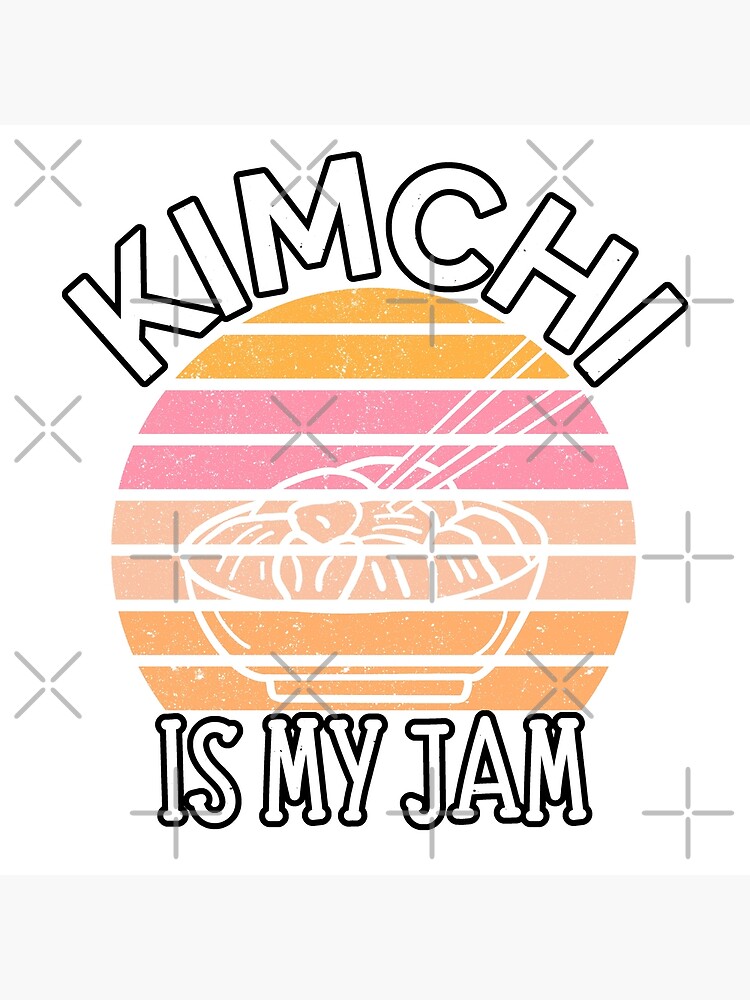This computer-generated illustration, possibly intended as a sticker design, features a central circular motif with a vibrant banded pattern of color stripes: two light orange stripes, two pink stripes, two peach stripes, and two coral-colored stripes. Each band is separated by clear white stripes. Superimposed on these colorful bands is a line-drawn bowl of kimchi with two chopsticks pointing upward to the right. The bowl itself is not filled with color but allows the background stripes to show through, creating a translucent effect. Above the circle, in block capital letters with a black outline and no fill, are the words "KIMCHI." Below the circle, partly obscuring the bottom two stripes, is a white square bearing the text "IS MY JAM" in similar block capitals with a black outline. Overlaying the entire image are numerous lightly grayed X-shaped symbols or hash marks, likely serving as a stylized watermark to prevent duplication.